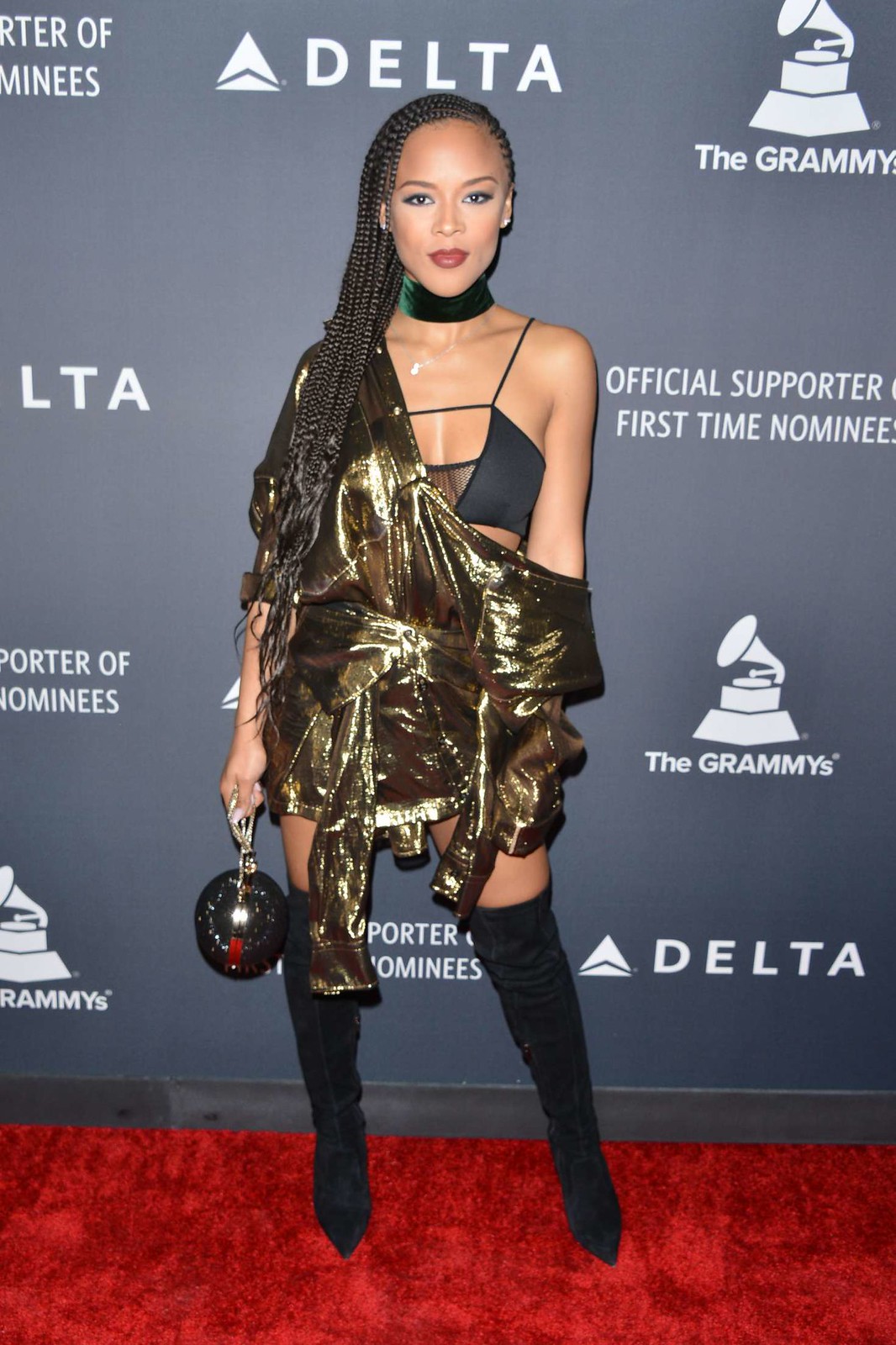In this captivating Grammy Awards red carpet photograph, a stunning young African-American woman of very fair skin and African heritage gazes confidently towards the camera. She sports long braided hair with elegant extensions, accentuating her beauty and youth. Around her neck is a striking green velvet choker, adding a splash of color to her ensemble. 

Her avant-garde outfit features an off-the-shoulder, short gold metallic tunic that highlights her décolletage, partially revealing a black bra beneath. A wide belt cinches her waist, complementing the glitzy vibe. In one hand, she clutches a unique, round black purse adorned with glitter, reminiscent of a small bowling ball, hanging from a delicate gold chain.

Drawing further attention to her bold fashion choices, she wears black, form-fitting thigh-high boots that reach just above the knee and culminate in sharp points. The backdrop is a gray wall adorned with white lettering and logos for Delta and the Grammys, emphasizing her presence at this prestigious event. She stands elegantly on the iconic red carpet, embodying both sophistication and avant-garde style.